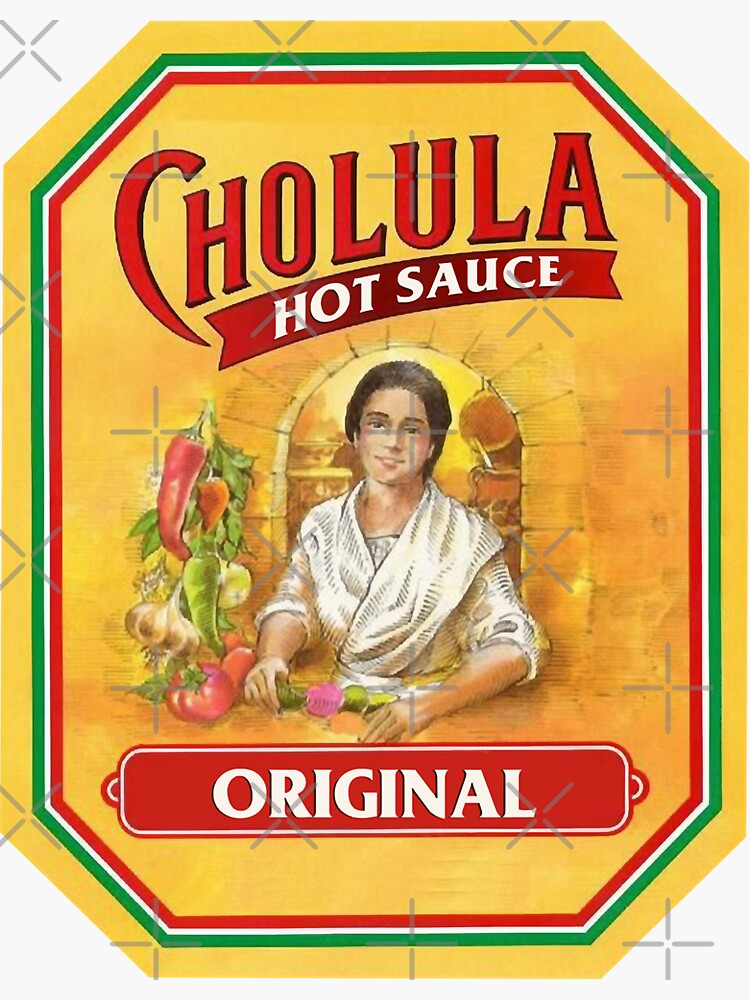This image features a promotional poster for Cholula Original Hot Sauce, uniquely designed with a rectangular base but with diagonally cut corners giving it an uneven hexagonal shape. The poster has a vibrant yellow background with a red and white text at the top that reads "Cholula Hot Sauce" and "Original" written at the bottom. At the center, there is an illustrated woman dressed in a white jacket, smiling while appearing to prepare vegetables and peppers, possibly for her signature hot sauce recipe. Surrounding her are various fruits and chili peppers, adding to the culinary theme of the image. Additionally, the entire poster has a subtle cross-shaped watermark and is bordered by a distinctive green, white, and red trim, completing the look of this eye-catching label.